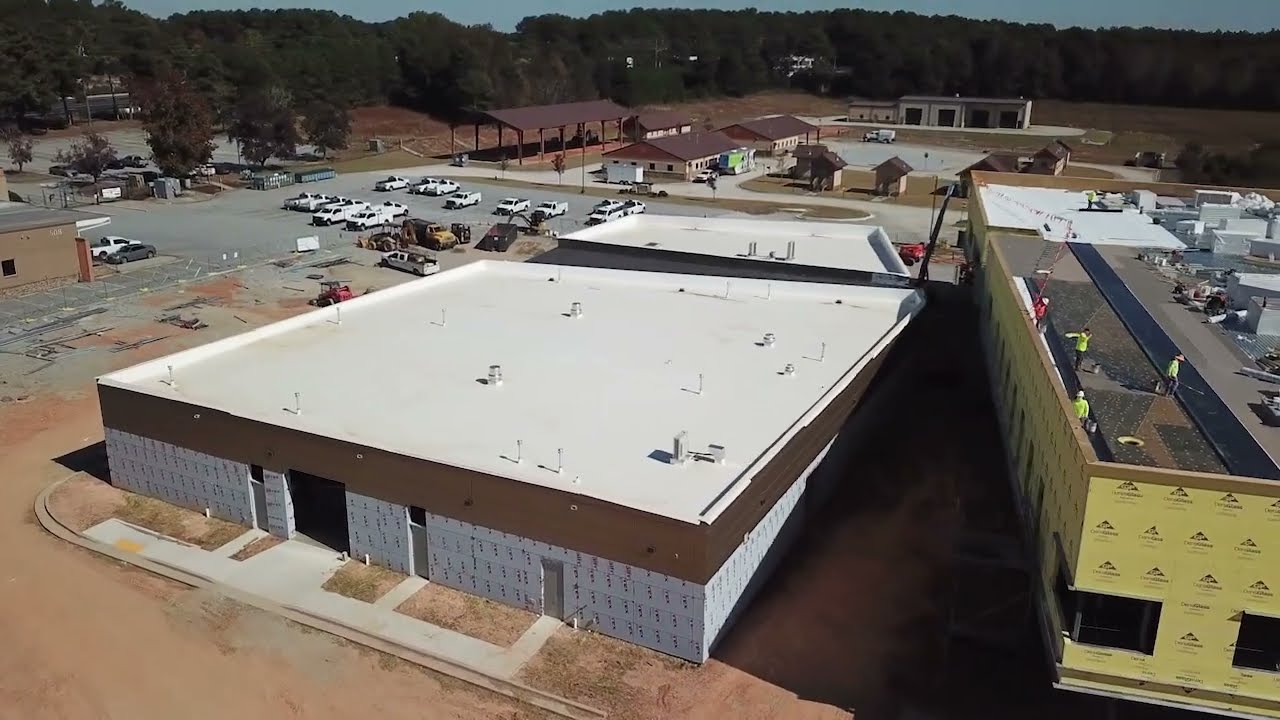This aerial color photograph captures a construction site with multiple buildings in various stages of completion. The foreground features a prominent large building with an unfinished exterior, wrapped in white Tyvek material, and topped with a flat, white roof. To its right, a two-story building is covered in a yellow wrapping, with several construction workers noticeable on the roof, distinguished by their high-visibility yellow shirts and gray pants, and one worker in an orange shirt. Scattered around them are construction materials, though fine details are difficult to discern due to the distance.

In the background, there is a parking lot filled with white trucks, likely belonging to the construction crew. Beyond the immediate construction area, a couple of smaller buildings with brown roofs and cream siding are visible. The wider landscape includes roads and pockets of green trees, giving a sense of an emerging urban or suburban development zone. The overall impression is of a dynamic, partially developed area with active construction and future potential.